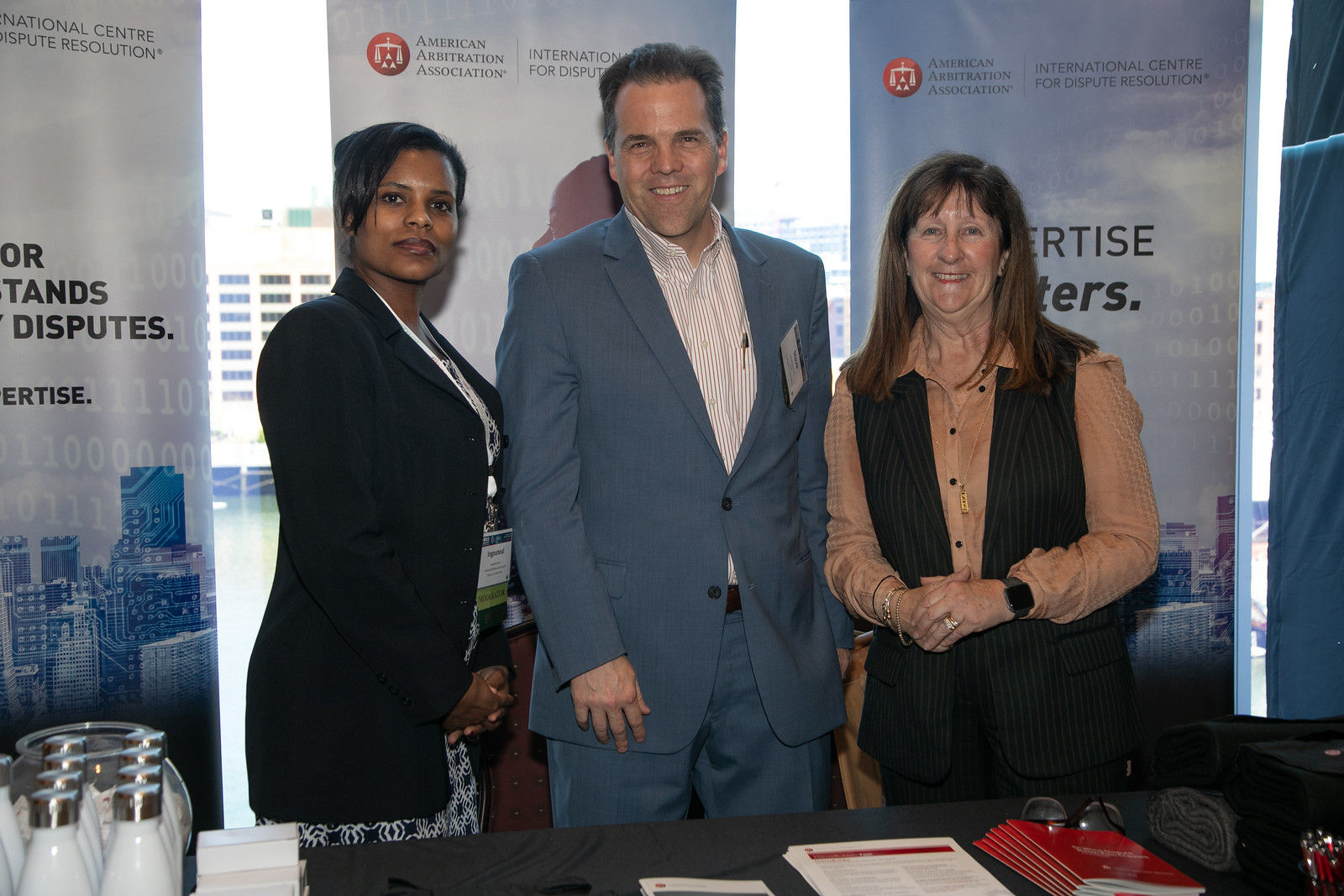Three individuals are posing for a photo in front of a small covered desk adorned with pamphlets and water bottles. The backdrop features banners with the logo of the American Arbitration Association and the International Center for Dispute Resolution, hinting at the event's theme. Centered is a man wearing a blue-gray suit, paired with a red and white striped shirt, and a visible employee ID on his left side. To his left stands a black woman in a black coat and a knee-length black and white checkered skirt. A blue lanyard hangs around her neck, and her hair is pulled back. To his right is a white woman dressed in a rust-colored long-sleeve blouse accented with black buttons, a black vest, and assorted jewelry including a black watch with a gray band. She stands slightly shorter than the black woman, completing the trio’s professional appearance.